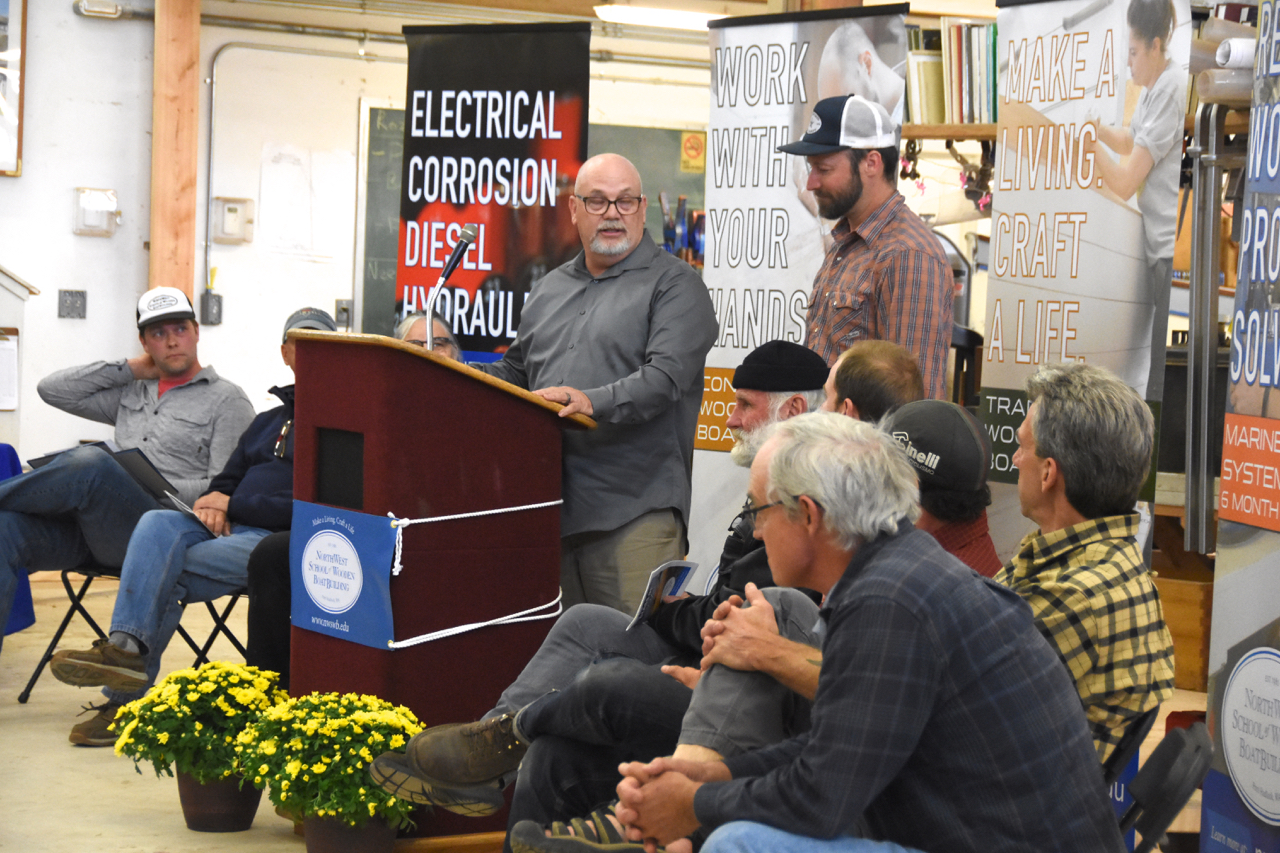In the photograph, an elderly man, approximately 40 to 50 years old, stands at a brown podium speaking into a microphone. He is bald, wears glasses and has a grey goatee. To his right, a man with a black beard, wearing a baseball cap and flannel shirt, listens attentively. Surrounding the podium are about eight men seated on chairs, some middle-aged to older, all focusing on the speaker. The setting appears to be a workers' union meeting, as suggested by the prominent blue banner and various other banners in the background. These banners feature phrases such as "Electrical, Corrosion, Diesel, Hydraulic," "Work with Your Hands," and "Make a Living, Craft a Life," indicating discussions about trade and electromechanical industries. Two pots of flowers decorate the front of the speaker's desk, adding a touch of formality to the scene.